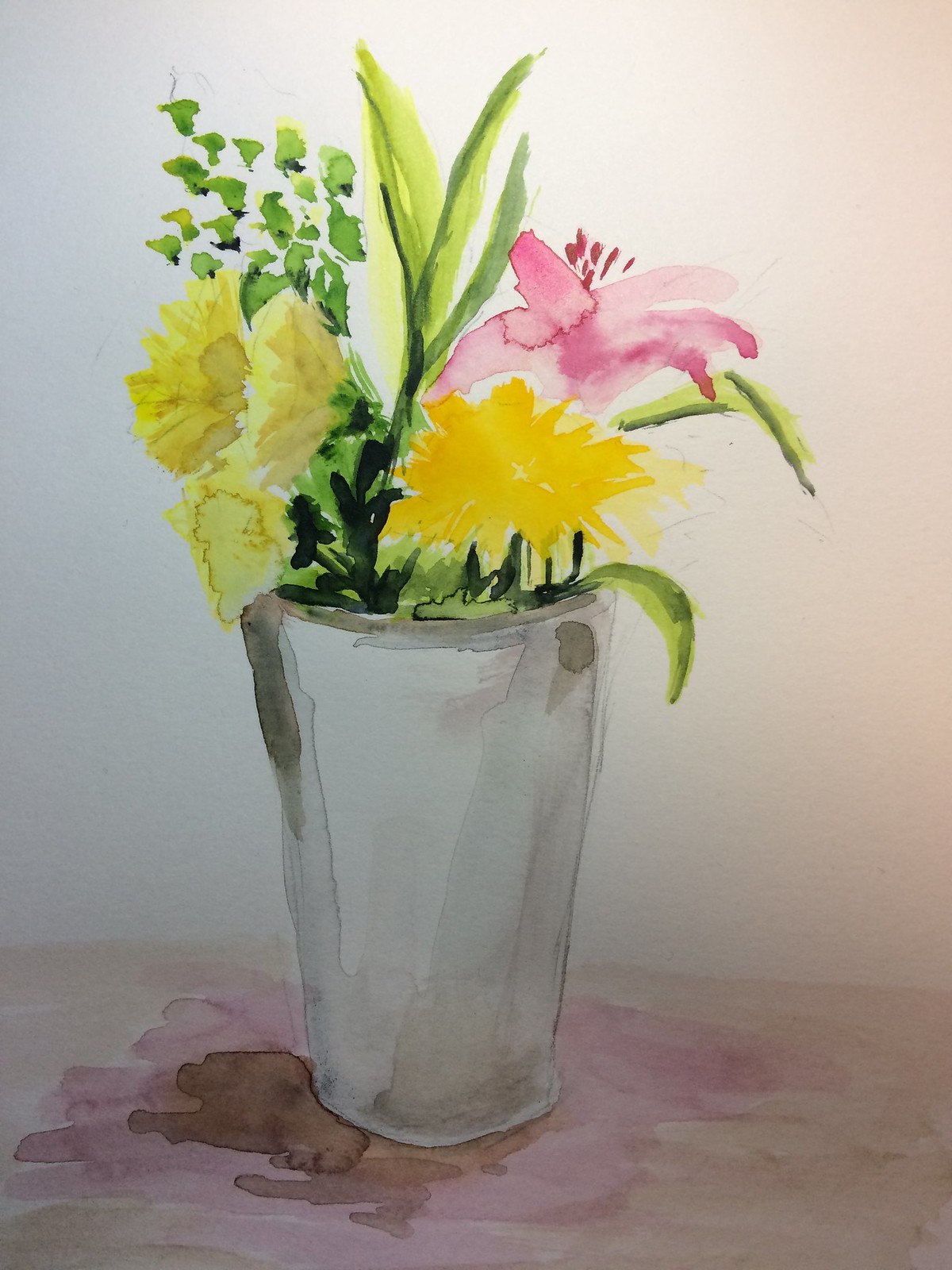The image is a detailed watercolor painting on a rectangular sheet of paper, depicting a white glass vase with a flared top, sitting on a red table. The vase contains a diverse array of flowers, including sunflowers, tulips in pink and white, yellow daffodils with green backs, and a pink orchid-like flower. There is also a unique red flower with bent green leaves that resembles a dandelion. Various shades of green and light green leaves, some narrow and long, others smaller, fill out the arrangement. The table surface beneath the vase is rendered in shades of brown, pink, and dark red, with some areas showing color bleeding, suggesting either dirt or artistic texture. Splashes of white and brown around the base of the vase add to the natural feel of the composition, enhancing the watercolor effect with hints of smudging and staining.